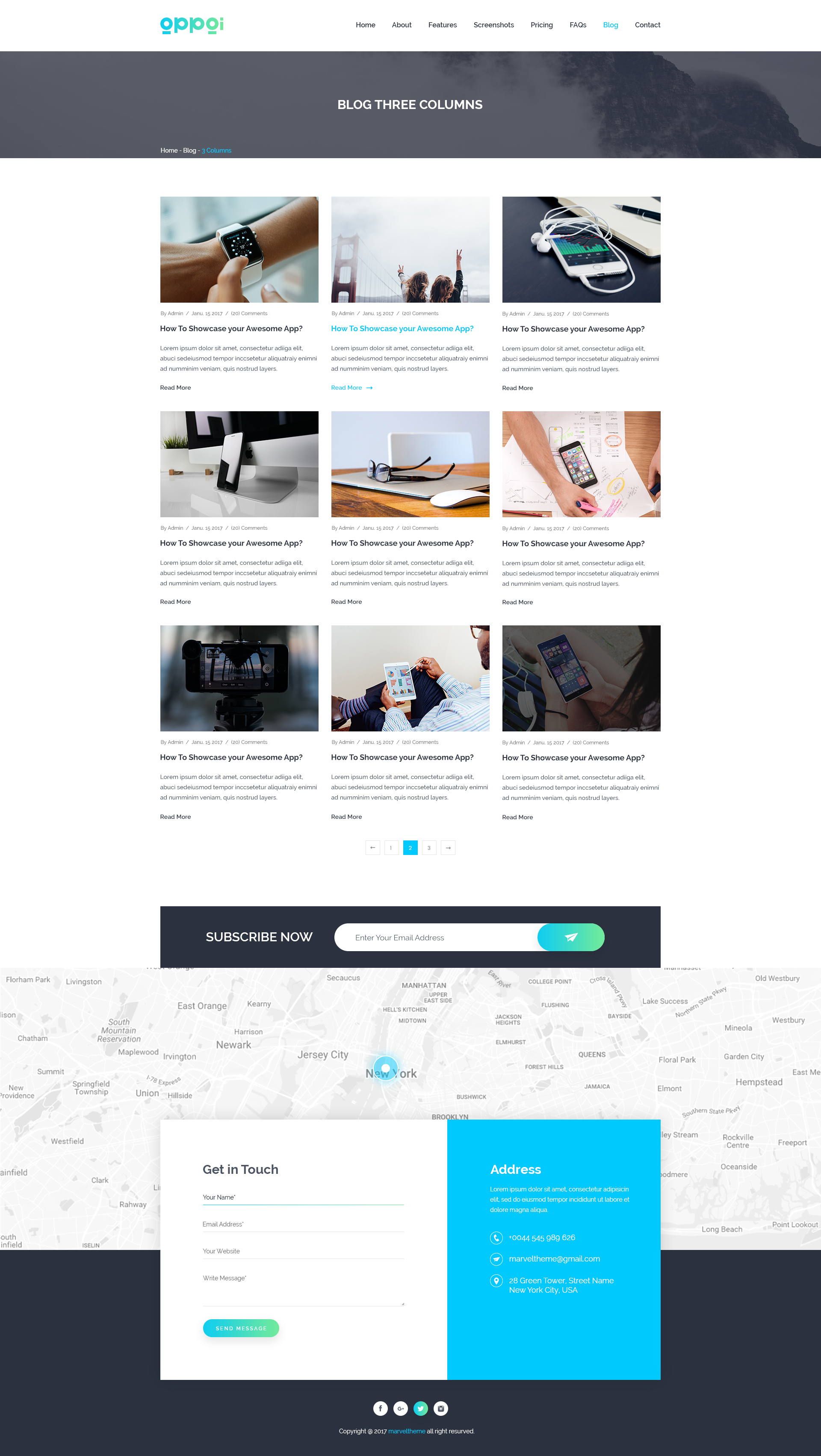This image is a detailed screenshot of a computer interface. At the very top of the screen, the header displays "OPPOI." Adjacent to the header are several selectable options, with the "Blog" option highlighted. Below the header, there is a prominent gray border labeled "Blog, Three Columns."

The main section showcases a grid of nine images arranged in three rows and three columns. Most images depict various smartphones or digital devices, with one notably featuring a smartwatch. Beneath this gallery of images is a "Subscribe Now" button alongside an input field presumably meant for users to enter their email addresses.

Toward the bottom of the screen is a map, likely indicating a physical location. Overlapping the map is a pop-up window titled "Get in Touch." On the right side of this pop-up, there is a blue box containing address details for contacting the company or service being displayed.

Finally, the footer of the interface is rendered in black, displaying social media icons for Facebook and Instagram, providing a means for users to follow or contact the organization through these platforms.